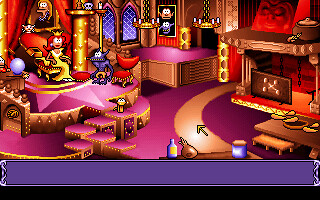The image appears to be a screenshot from a retro, pixelated fantasy-themed video game, featuring vibrant colors such as pinks, oranges, reds, and yellows. At the center of the scene, a princess or queen, with long red hair and a yellow crown, is seated on a heart-shaped throne at the top of purple stairs on a large purple platform. She is donning a long yellow dress. To her right stands a purple creature characterized by a long purple snout with a red nose, white eyes, and jagged teeth. Another seat is nearby, possibly for the creature. The surroundings suggest an opulent castle or palace room, with intricate details such as chandeliers and stained glass. On the far right is a fancy fireplace adorned with a red face figure above it. The floor is covered with a pink carpet, further adding to the grand and ornate atmosphere. At the bottom of the image, there is a purple text box with no text in it, suggesting potential dialogue or commands within the game.